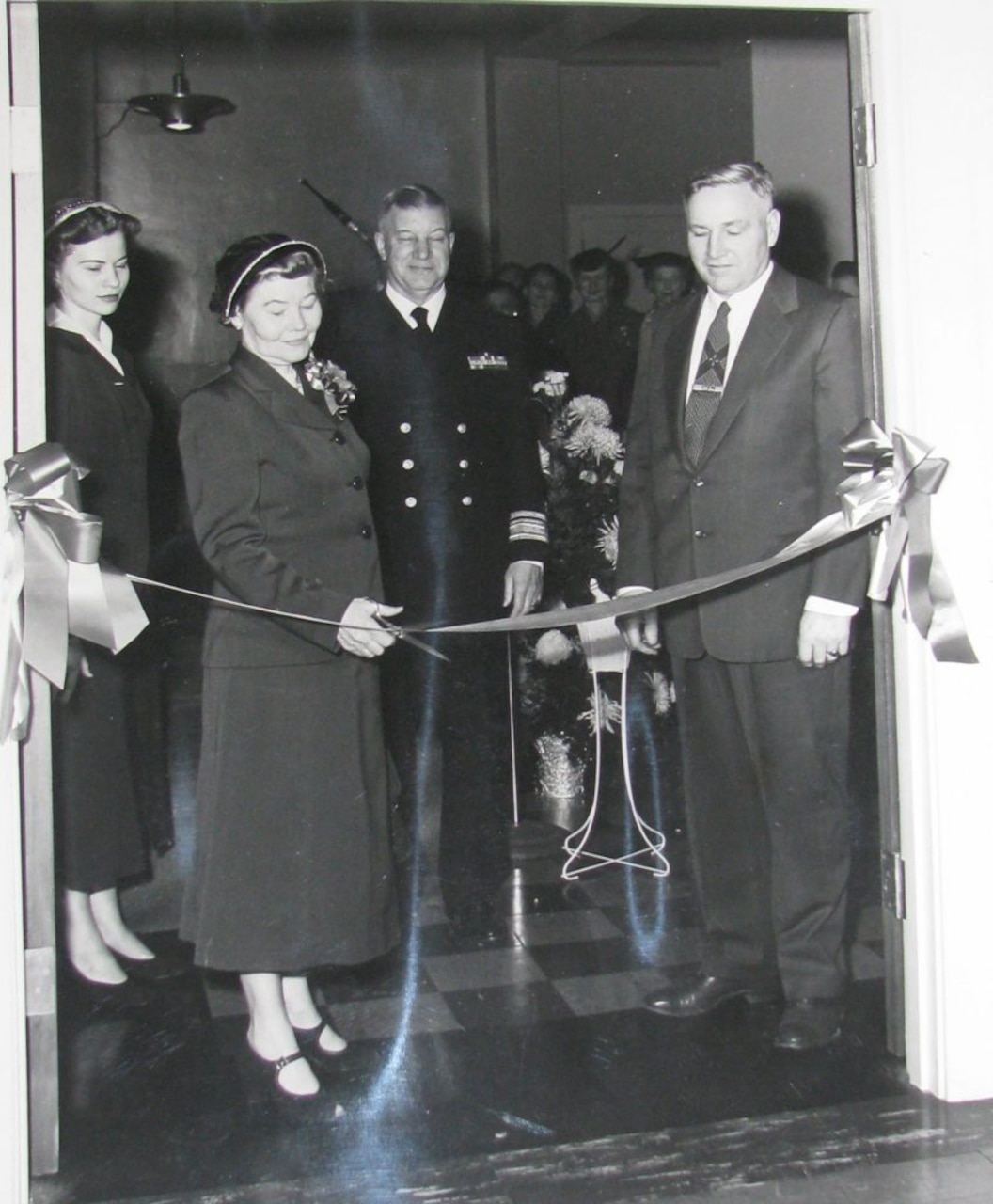The black and white photograph captures a ribbon-cutting ceremony at a double-door entrance framed in white wood. The central focus is a woman dressed in a dark, elegant gown, adorned with a hat and a flower on her chest, holding a pair of scissors poised to cut the ribbon draped across the entrance. Surrounding her are key figures, including a man in a black suit with a white shirt and tie on her right, and another man to his left dressed in a naval uniform. To the left of the naval officer stands another woman in a similar long dress and hat. They stand on a checkered white and black tiled floor, with a small display of flowers placed near the naval officer. In the background, a crowd of people, some wearing hats, watch attentively, their expressions hinting at an air of celebration illuminated by the camera's flash. The scene is bustling with a mix of spectators filling the space beyond the entrance, adding to the photograph's historic ambiance.